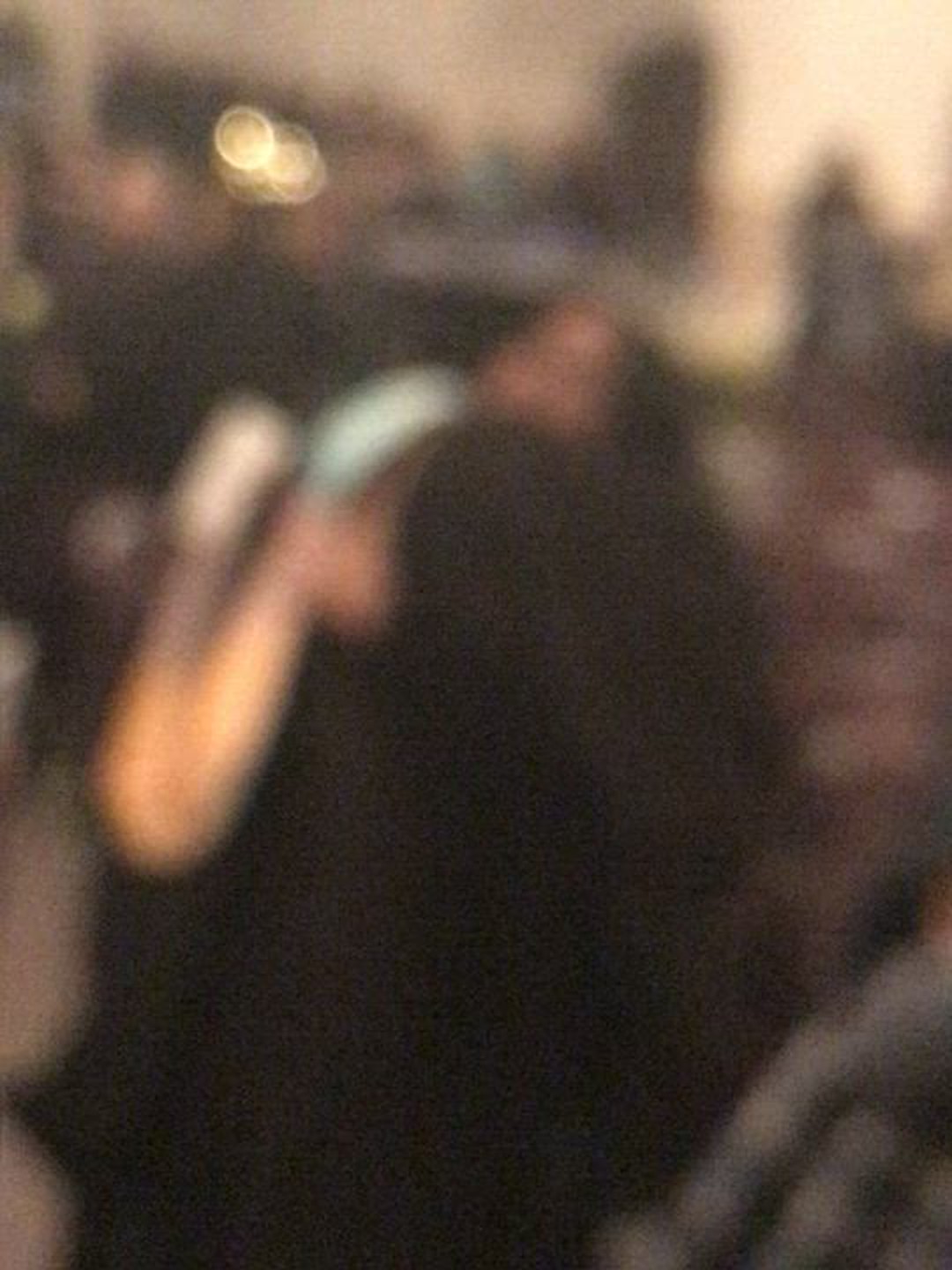This very blurry color photograph depicts a scene with various shades of brown and white, making it challenging to identify objects clearly. In the upper left-hand corner, there is a light source illuminating part of the image beneath a dark brown area. The center of the image is dominated by darker and black tones, surrounded by gray edges. Part of a person’s face is visible, obscured by the blur, with dark hair and dark clothing. Their arm is bent upward, culminating in a white area possibly representing a hand, with a skinny gray section underneath. In the upper right-hand corner, another light area can be seen.

Appearing in the bottom middle of the frame, a brown object that could be a handbag or purse is distinguishable, with shimmering golden handles visible across its top. The scene hints at a complex background that includes elements like diagonal gray beams in the bottom right and what may be a brown rectangular door towards the upper portion. This photograph might capture two individuals in dark graduation robes embracing, suggestive of an outdoor graduation event filled with movement, chairs, and a spotlight that perhaps hints at a post-ceremony atmosphere. The objects and figures within the photo are obscured by intense blurriness and out-of-focus details, making it open to varying interpretations.